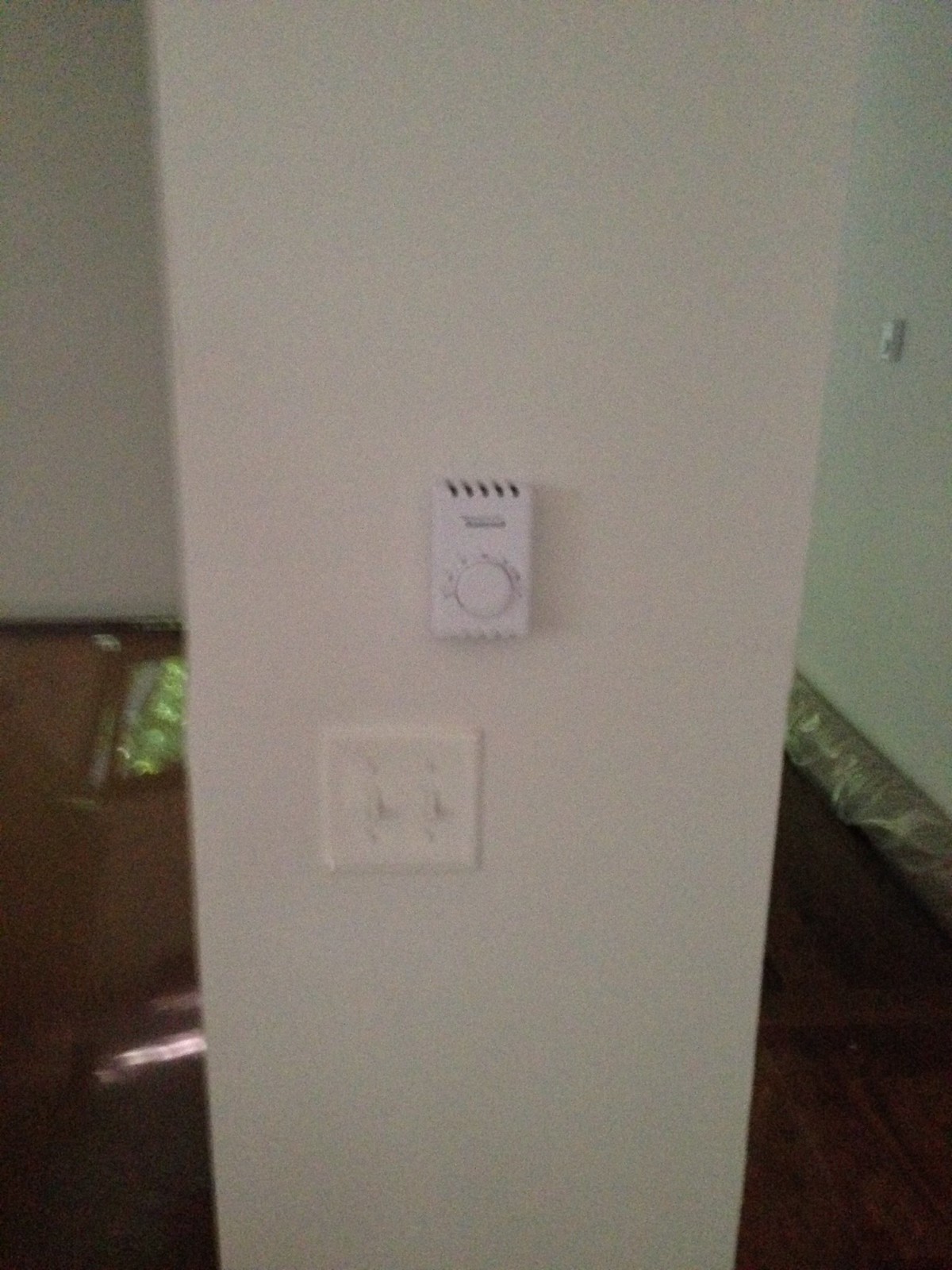The image depicts a section of an interior wall in a building. The wall is painted white and contrasts sharply with the wooden brown floor beneath it. This short, narrow wall serves as a divider between two separate areas within the space. Mounted on the wall is a white light switch panel featuring two toggle switches, each secured with two screws. Positioned above the light switch is a white device with a central dial surrounded by numbers, likely a thermostat. To the right, partially visible in the adjoining area, is another wall-mounted device with a similar dial. The overall image is blurry and slightly out of focus, making details less distinct. The left portion of the room contains a green object on the floor, but it is too blurry to identify clearly.